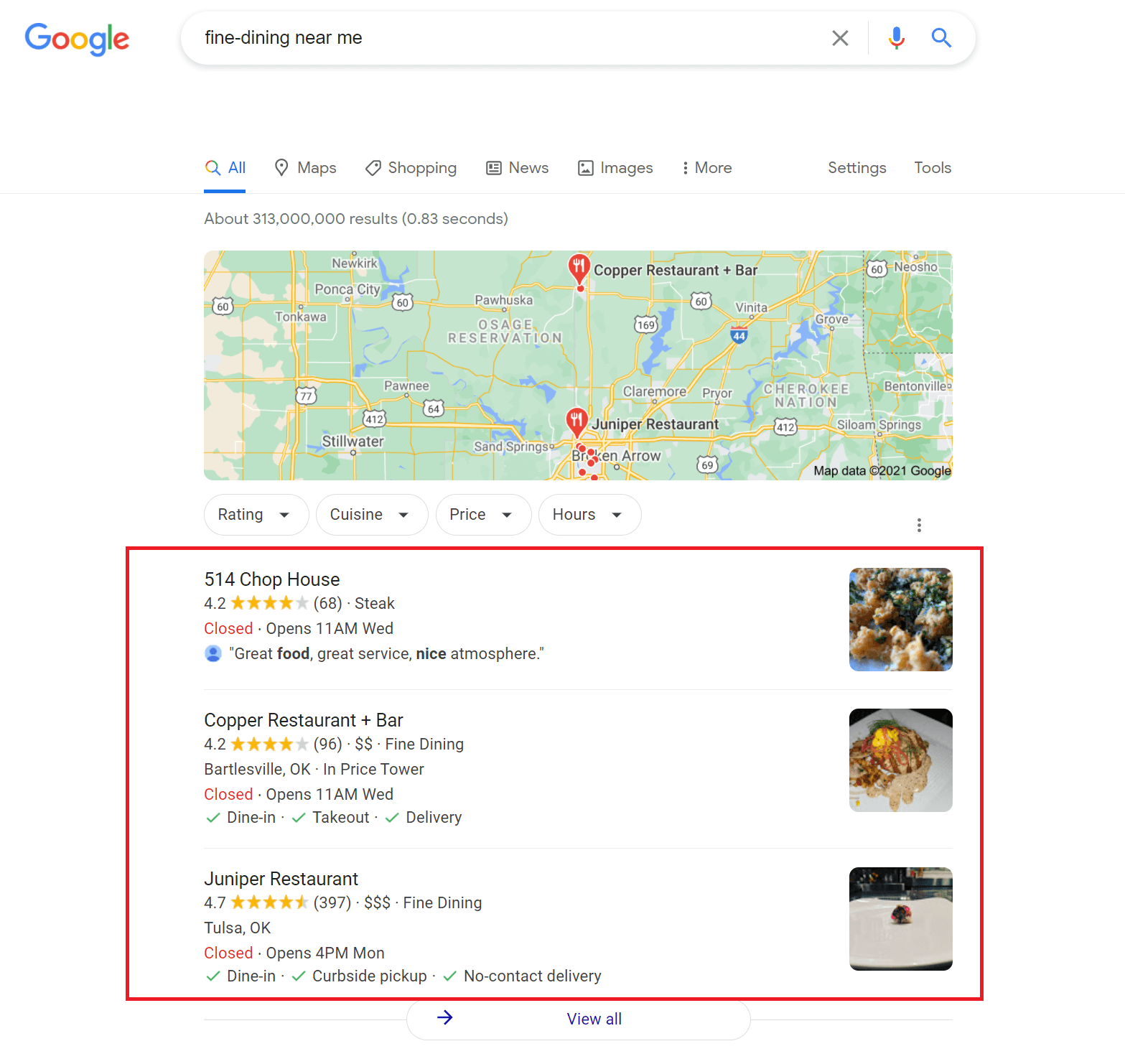The image features a Google search result page for the query "fine dining near me." Displayed prominently at the top, the search bar contains the query, with tabs for "All," "Maps," "Shopping," "News," "Images," "More," "Settings," and "Tools" lined up below it. Google states there are approximately 313 million results, which were retrieved in 0.83 seconds. 

Just beneath this, a map adorned with several red location pins pinpoints various dining options. Under the map, filters such as "Rate and cuisine," "Price," and "Hours" are visible, aiding in refining the search.

Enclosed in a red rectangular box beneath these filters is a list of specific restaurant results:
1. **514 Shophouse**: Rated 4.2 stars based on 68 reviews. It is known for steak but is currently closed and will reopen at 11 a.m. on Wednesday. Descriptive phrases include "great food," "great service," and a "nice atmosphere."
2. **Copper Restaurant and Bar**: Also rated 4.2 stars, with 96 reviews. Located in Bartlesville, Oklahoma, specifically in Price Tower. It's described as a fine dining establishment offering dine-in, takeout, and delivery options. It is currently closed and set to open at 11 a.m. on Wednesday.
3. **Juniper Restaurant**: This establishment holds a 4-star rating, but no further details are provided within the captured image.

The detailed search results give potential diners a quick overview of their highly rated and convenient dining options.